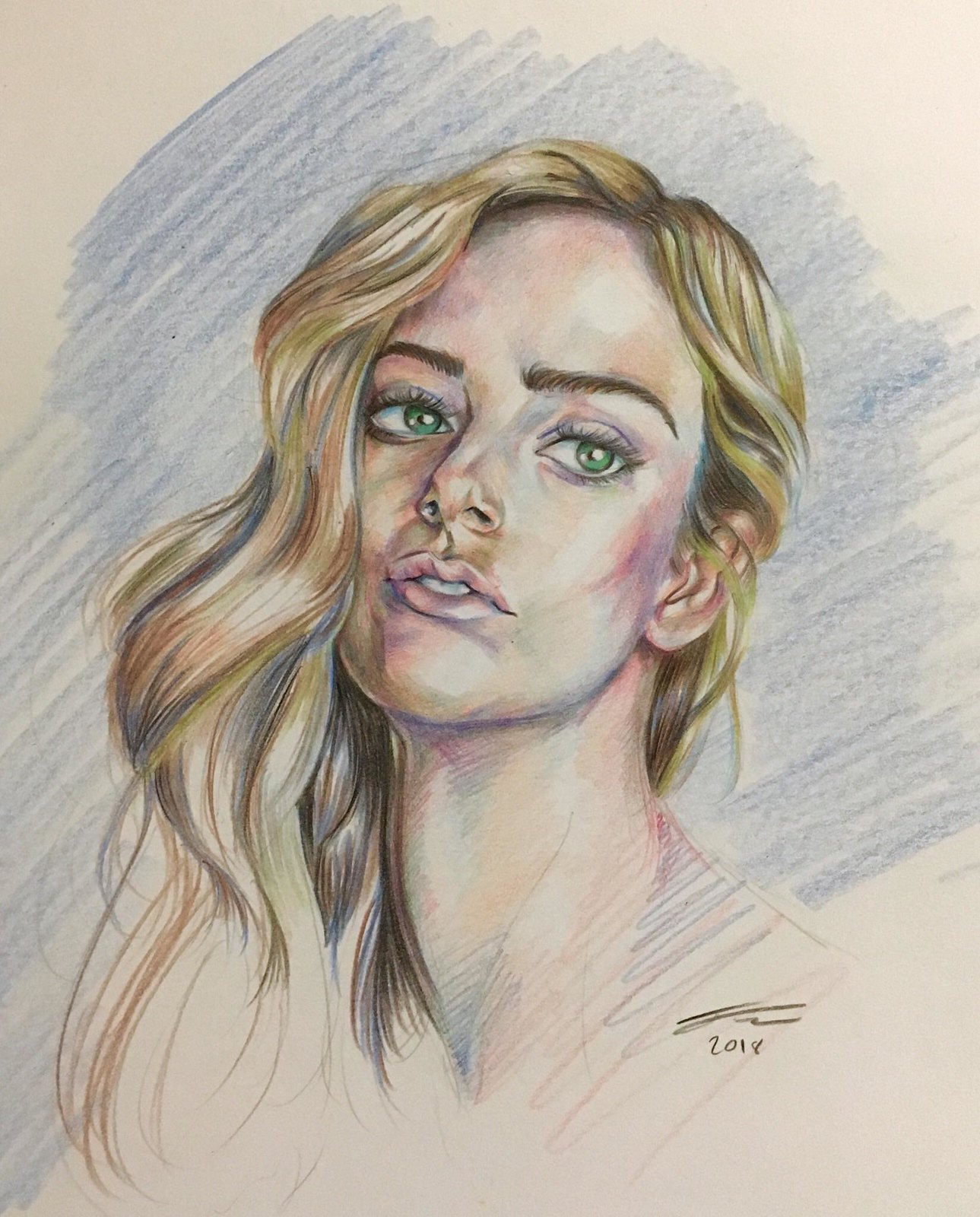This detailed colored pencil drawing depicts a young woman of European descent with blonde hair. The subject is gazing thoughtfully to her left. The artist has meticulously rendered her eyes, lips, and nose with striking precision, showcasing an impressive level of detail. Set against a blue background, the drawing exudes an ethereal quality. A signature in dark red ink, marked with the year 2018, is inscribed in the bottom right corner, suggesting it may be a self-portrait.